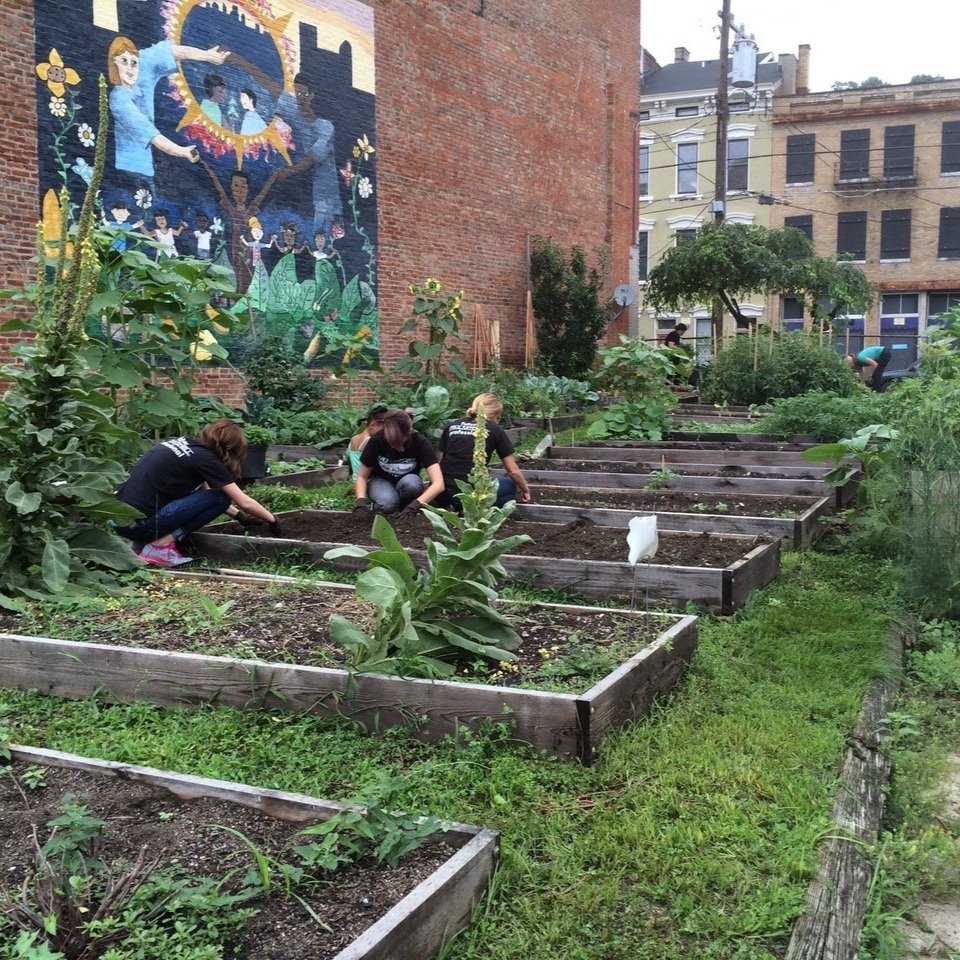This vibrant photograph captures a bustling urban community garden, framed by a backdrop of red brick buildings and apartment complexes typical of a cityscape. The central focus is a group of young adults, likely college or high school students, diligently tending to several rectangular wooden raised garden beds. The dark brown soil contrasts with the greenery of various plants – sunflowers, tall wildflowers, and edible herbs and shrubs. 

Five individuals, mostly dressed in black t-shirts with one in a green tank top, kneel and crouch, their gloved hands immersed in planting seeds or digging. The scene suggests a collaborative project, possibly part of a class or community initiative.

To the left, a large brick building sports a colorful mural depicting children and adults in vibrant scenes, including a gold ring with dancing figures, adding artistic flair to the urban environment. The mural features a skyline silhouette and a woman with her arms outstretched, symbolizing growth and community spirit. The setting is completed with fence lines and telephone poles, emphasizing the garden’s placement within a bustling city neighborhood.